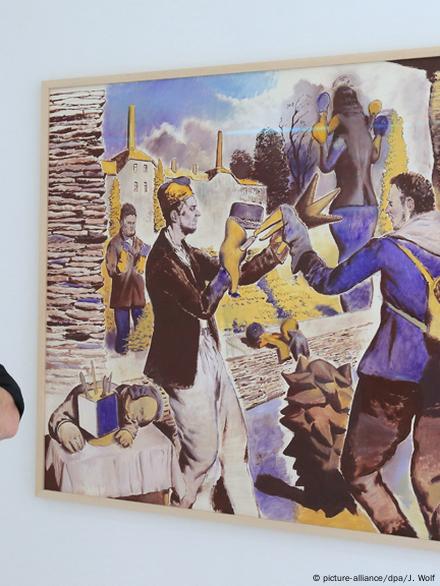This photograph captures a detailed painting displayed on a light blue wall, with part of a person's elbow visible in the left corner. The painting is encased in a thin, beige-colored wooden frame. The artwork portrays a complex scene, with several distinct elements:

At the center, two men appear to be engaging with each other. The man on the right is dressed in a purplish-blue coat and brown pants, wearing a yellow backpack while reaching out towards the other man. He holds an object, possibly a bird-like star. The man on the left is clad in a brown jacket, white pants, and a yellow hat, and seems to be trading or interacting with the other individual.

In the foreground, a man wearing a brown jacket and blue pants leans against a table, appearing to be asleep with a book beside him. Another figure, also in a brown jacket with blue pants, stands against a brick wall nearby.

The background of the painting includes a picturesque depiction of old European architecture, featuring stone walls, buildings, statues, and some greenery under a blue sky with white clouds. Additionally, there are some indistinguishable objects and structures within the scene, adding to its intricate nature.

At the bottom of the painting, a footnote reads "copyright picture - alliance / dpalj.wolf."